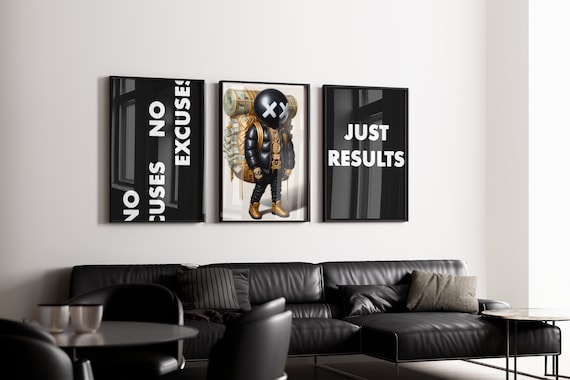The image depicts a very modern and chic living room or break room with a stark black and white theme. The room features pristine white walls, providing a clean contrast to the large black leather couch adorned with a mix of black and gray throw pillows. Adjacent to the couch is a small side table. Situated further into the room is a round table with a sleek silver top, surrounded by three black leather chairs, with two stainless steel mugs placed on its surface. Above the couch, three distinct black and white posters are neatly aligned. The first poster, with "no excuses no excuses" written in white on a black background, is displayed sideways. The middle poster features an artistic depiction of a humanoid figure with a large black head marked by two white X's over the eyes, dressed in a black leather vest, black pants, and brown boots, and carrying a substantial pack. The third poster reads "just results" in white text centered on a black background. The overall atmosphere of the room is enhanced by daylight streaming in from an unseen window, emphasizing the room's clean and modern aesthetic.